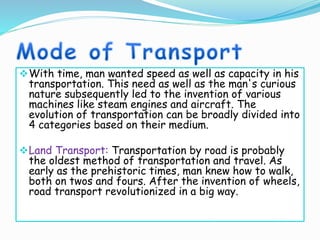The image is a small, square slide with no surrounding border, featuring a detailed explanation about the history of transportation. At the top of the slide, there's a curved, blue-shaded wave design against a white background. Below this wave, the title "Mode of Transport" appears in blue Comic Sans font. Encased in a light blue outlined box are two diamond-shaped bullet points. 

The first bullet point reads: "With time, man wanted speed as well as capacity in his transportation. This need, along with man's curious nature, subsequently led to the invention of various machines like steam engines and aircraft. The evolution of transportation can be broadly divided into four categories based on their medium."

The second bullet point, starting with the title "Land transport" in purple text followed by black text, states: "Transportation by road is probably the oldest method of transportation and travel. As early as prehistoric times, man knew how to walk both on twos and fours. After the invention of wheels, road transport revolutionized in a big way."

The overall content provides a concise yet comprehensive overview of the progression of transport methods, emphasizing land transport and the significant advances following the invention of the wheel.